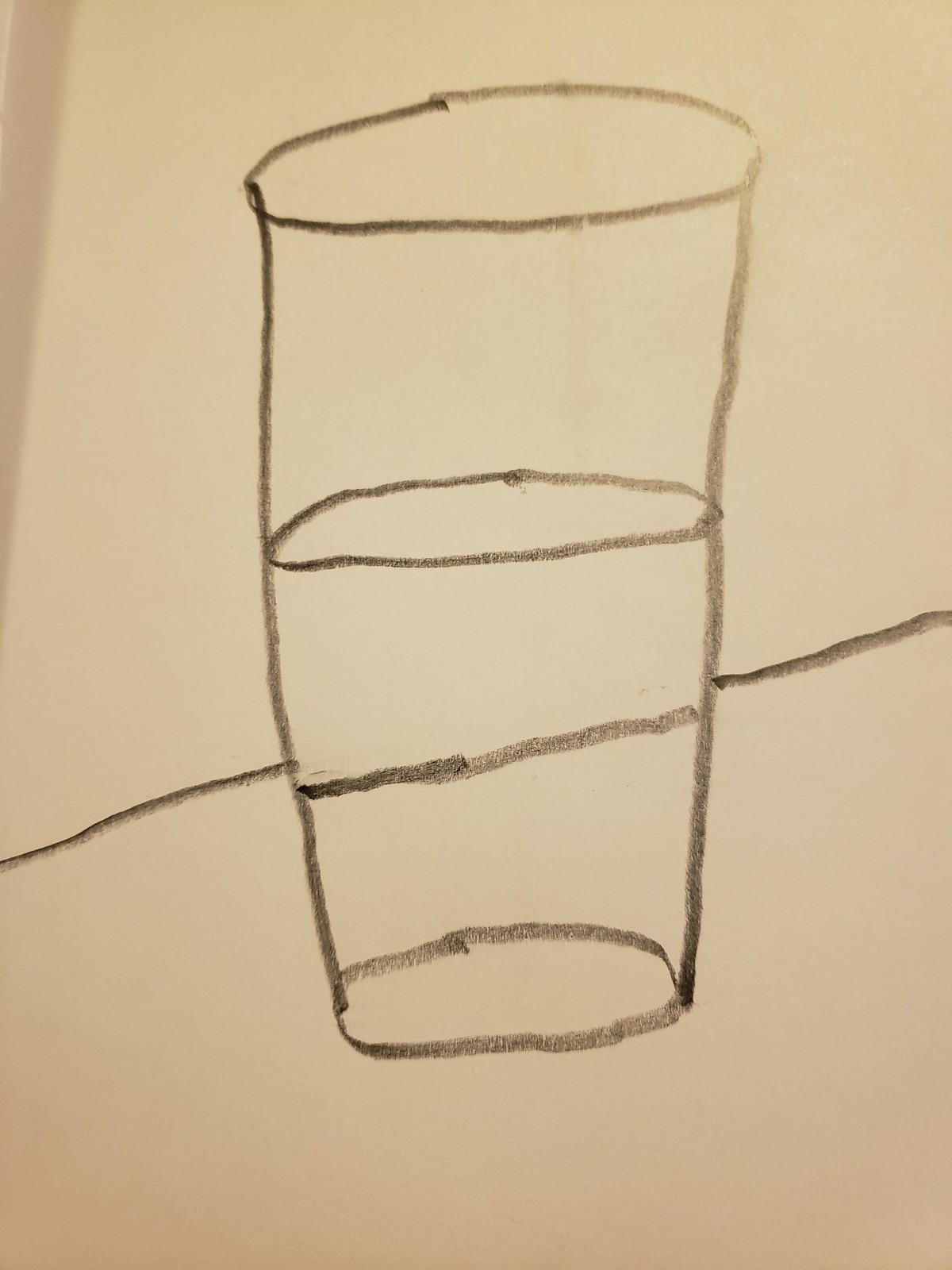A black and white photograph of a simple, rudimentary drawing, possibly done with pencil or pen, features a cup filled with water. The minimalist sketch is characterized by basic line work, devoid of any shading or intricate details, suggesting it may be the effort of a beginner artist.